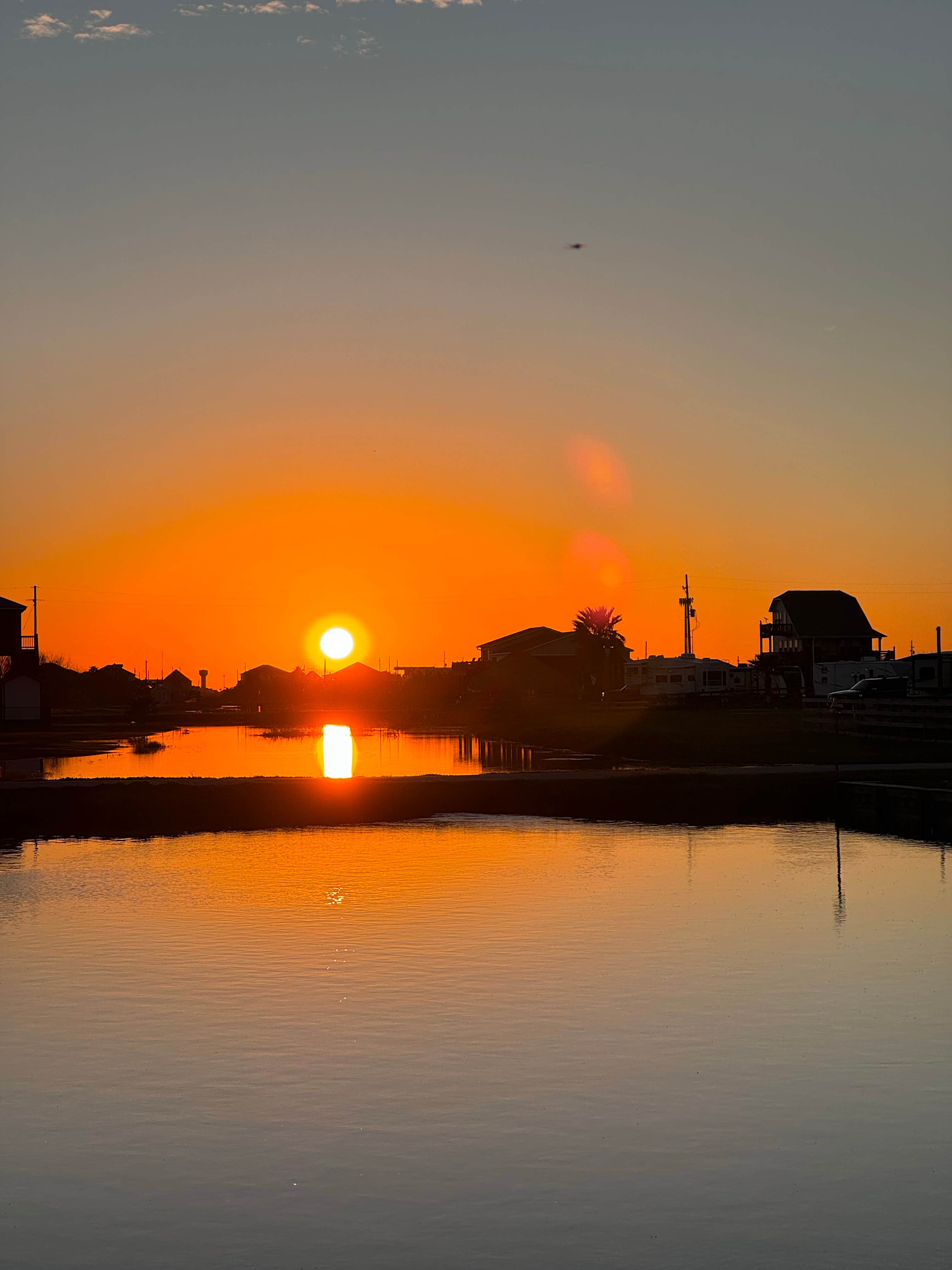The photograph captures a breathtaking sunset over a narrow canal lined with houses and buildings on both sides. The viewer's perspective is from above the water, which is tinted gray-blue and reflects the bright orange and yellow hues of the setting sun. The sun sits just above the horizon, casting a warm glow that gradually cools as it extends upward into a light gray, then darker blue sky. Toward the upper part of the image, a few clouds are visible, adding texture to the expanse. There is a bridge or walkway crossing the water, and while it's difficult to discern details due to the dimming light, some parked cars and sparse trees are noticeable. The overall scene embodies the serene transition from day to night in a picturesque town beside the water.